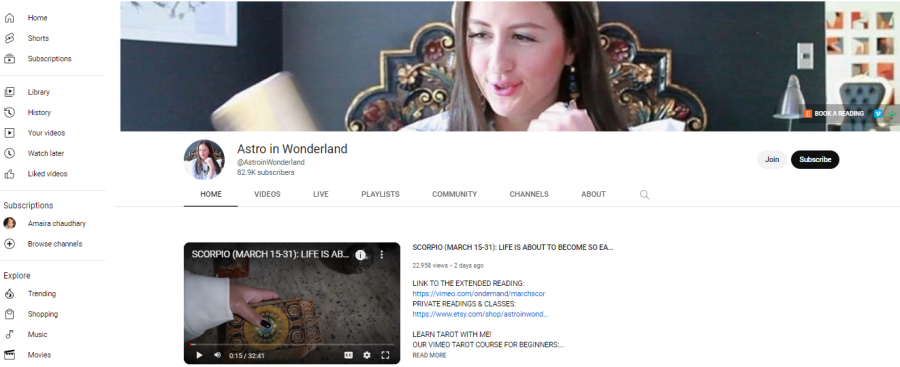This image is a screenshot of a YouTube channel page. On the left side, there's a white sidebar. Dominating the top right section is a banner featuring a photograph of a woman with brown hair. The background of the banner is an ornate dark gray wall adorned with a golden floral design. Below this banner, the channel name "Astro in Wonderland" is displayed, accompanied by the handle "@AstroinWonderland" and the subscriber count of 82.9k.

Underneath the channel name and subscriber information, there is a navigation menu featuring tabs for Home, Videos, Live, Playlists, Community, Channels, and About. Beneath this menu, a video player is visible against a light-colored background, likely indicating that the page has an overall light theme.